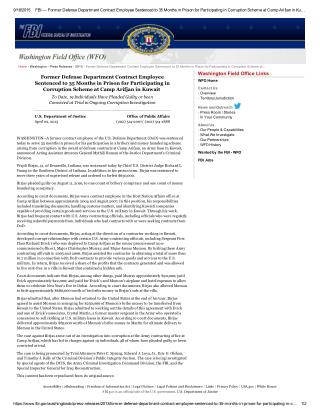The image is a screenshot of a website, but most of its text is too small to read clearly. At the top of the image, there's a gray search bar typical of many websites. To the left of the search bar, there appear to be initials "FB" and an employer identification number, indicating the source of the website. 

Below the search bar, there's a blue navy-colored banner featuring the initials "FBI" alongside a congressional seal in yellow and blue. The banner has text that reads: "Washington Field Office prepares the Defense Department to conduct employee service after 33 months in prison for participating in a campaign scheme in Kuwait."

The rest of the text in the image is too small and illegible.